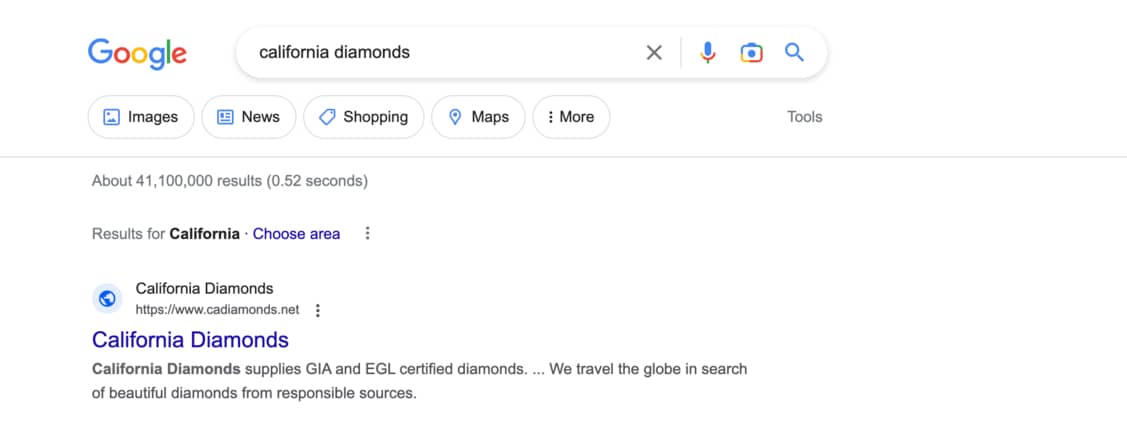This image showcases a cropped Google search results page. In the upper left corner, the iconic Google logo is prominently displayed, featuring the letters 'G' in blue, 'O' in red, 'O' in yellow, 'g' in blue, 'l' in green, and 'e' in red. To the right of the logo, the search bar shows the query "California diamonds", accompanied by a clear box 'X' to its right, a microphone icon for voice search, a camera icon for image search, and a blue magnifying glass icon, which acts as the search button.

Below the search bar, various tab options are visible, including "All," "Images," "News," "Shopping," and "Maps." To the right, a tools menu is labeled in light gray text. Beneath these tabs, the search results indicate approximately 41,100,000 results found in 0.52 seconds. 

The first search result is highlighted under the header "Results for California diamonds." The recommended link is www.cadiamonds.net, which leads to the California Diamonds homepage. The description beneath reads, "California Diamonds supplies GIA and EGL certified diamonds. We travel the globe in search of beautiful diamonds from responsible sources."